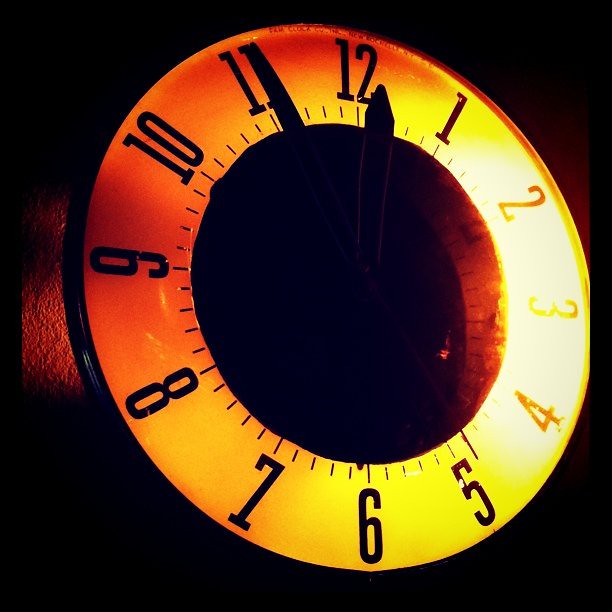This image captures an angled, up-close view of an illuminated clock face, prominently featured on a wall that appears to be textured and possibly concrete. The surrounding environment is extremely dark, adding dramatic contrast emphasized by the clock's illumination. The clock itself is round and large, with a black center that starkly contrasts the brightly lit outer ring which glows with hues of orange and yellow. This glow is most intense around the numbers 2, 3, and 4, making these parts of the clock particularly striking. The clock shows the time at 11:55, with the short hand at the 11 and the long, skinnier minute hand approaching the 12. Surrounding the clock face, the numbers are large and black, with four small black slashes between each numeral marking the minutes. Distinct shadows cast from the clock's light fall against the wall, enhancing the mysterious and dim ambiance of the room.